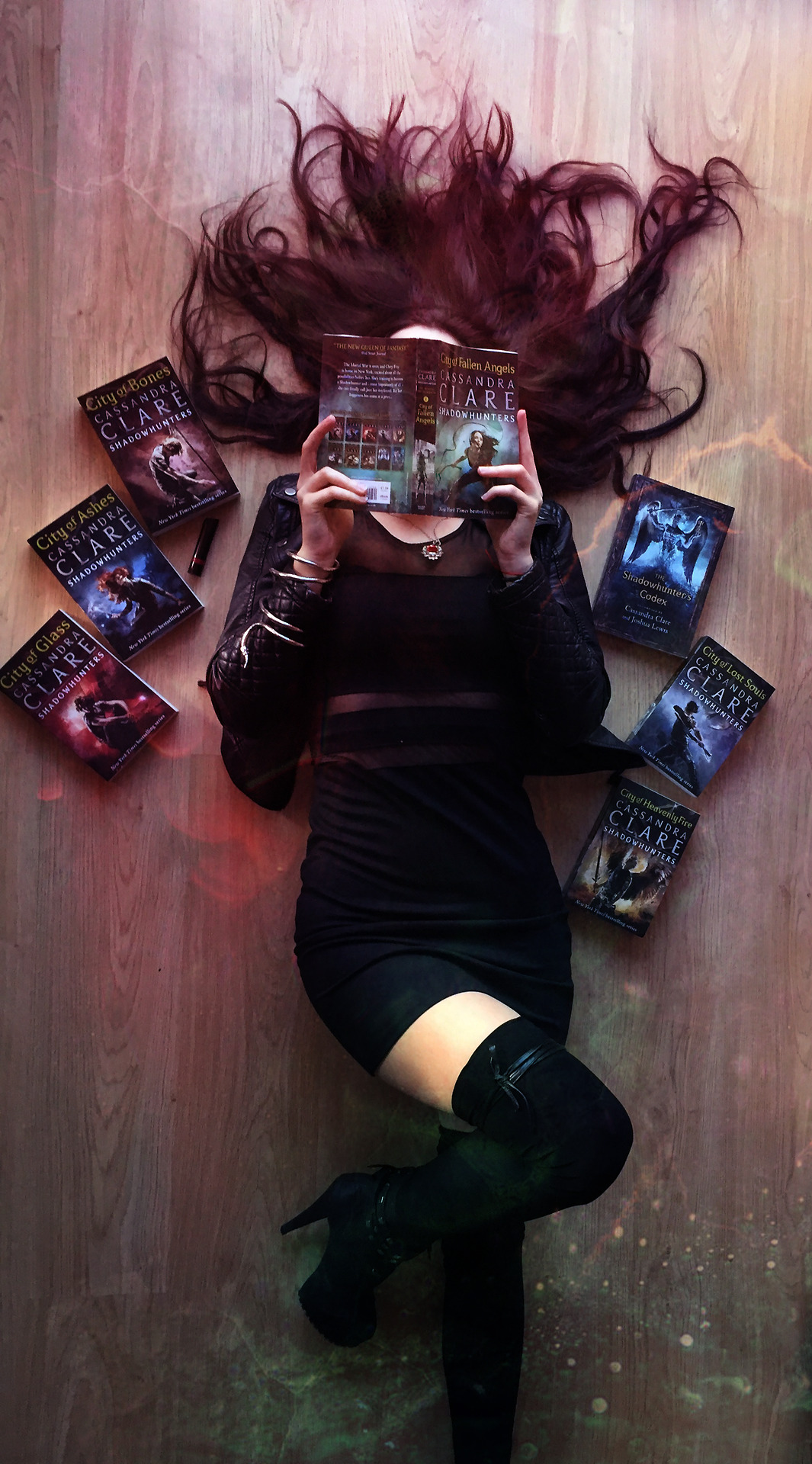This overhead color photograph captures a woman of white ethnicity lying on her back on a brown hardwood floor that shimmers with a faint green light near the bottom. The woman, dressed in a nearly mini black dress and thigh-high black stiletto boots, has her richly textured hair splayed out in a reddish-black fan behind her. A red pendant necklace adorns her neck, and a silver snake bracelet graces her right wrist. Her face is hidden behind an open book titled "City of Fallen Angels" by Cassandra Clare. Surrounding her are six other books by the same author, laid out on either side: "City of Glass," "City of Ashes," "City of Bones," "The Shadowhunter's Codex," "City of Lost Souls," and "City of Heavenly Fire." The overall scene emphasizes an immersion in literature, with the titles clearly readable and creating a thematic focus on Clare's works.